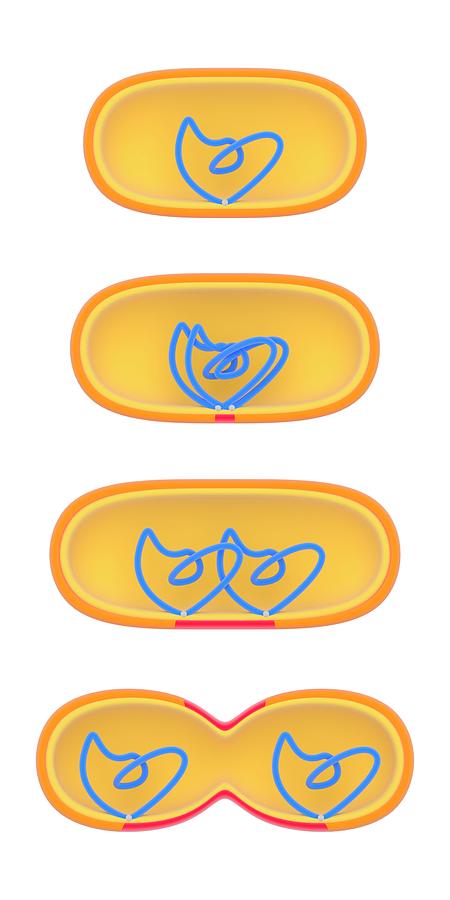The image displays a series of four progressively changing, oval-shaped objects arranged vertically from top to bottom. Each object transitions from a single, light orange oval with a yellow outline and a darker orange border to a figure-eight shape at the bottom. Inside each oval is a bright blue squiggly line resembling a heart. 

- In the topmost oval, there is a single blue heart-shaped squiggle.
- The second oval below it is slightly elongated and contains two overlapping blue heart shapes with a thin red boundary at the bottom.
- The third oval is even more elongated, and the overlapping blue hearts are positioned side by side, with the red section at the bottom becoming more prominent.
- The fourth and final object has split into a peanut or figure-eight shape with orange segments joined in the middle and separated blue hearts in each segment. The red outlines now cover the top and bottom of the object, suggesting a complete division.

This visual sequence perhaps symbolizes stages of development or division, similar to cell division diagrams in biology, where each phase shows further separation and differentiation of elements within the oval shapes.